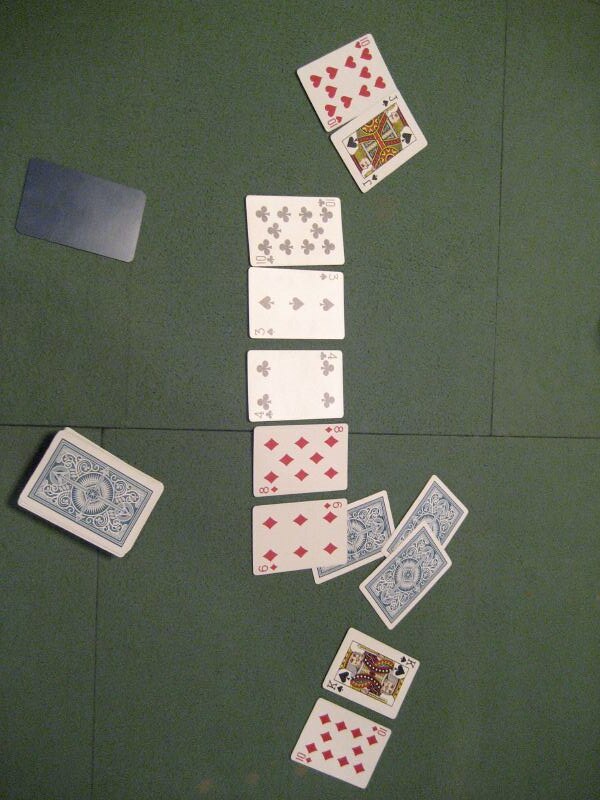The image provides a bird's-eye view of a green card table, possibly composed of four smaller tables pushed together. This configuration suggests a versatile table that can accommodate various card games. The table is cluttered with several cards, indicating an ongoing game. The picture appears to be tilted sideways, requiring viewers to tilt their heads right for proper orientation. 

On the left side of the image, there's a 10 of Hearts and a Jack of Spades. Nearby, a row of five cards includes the 10 of Clubs, 3 of Spades, 4 of Clubs, 8 of Diamonds, and 6 of Diamonds. Below the 6 of Diamonds, three cards are face down, with one directly underneath it and two adjacent. To the right, another set of cards includes the King of Spades and the 10 of Diamonds. Below this row, there is a single card without any back design, appearing as an end card rather than a joker. Additionally, there's a stack of cards featuring a blue and white scrollwork cross pattern, suggesting a standard card deck design. 

The scene captures the essence of a card game in progress, though the specific game remains unidentified.